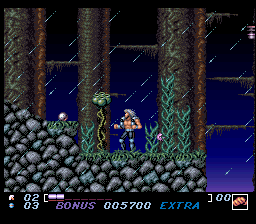In the bottom left corner of the image, there's a bar displaying "0-2." Adjacent to it, a device shows "0-3," and a purple bar is visible with two sections activated, possibly representing some sort of status or progress. A black area in the bottom left has a purple bonus indicator reading "0-0," "5-7," "0-0." Additionally, a blue section labeled "extra" is present, and a red section displays "0-0." Lights illuminate the scene, revealing what seems to be a stone wall adorned with rocks. The top of the wall appears patchy, with some areas having vines and ponds entwined, giving an impression of a lush environment. Moss-covered, lighter brown trees with sprawling branches are depicted, with raindrops falling gently. Central to this serene scene stands a figure with white hair, adding a human element to the natural setting.